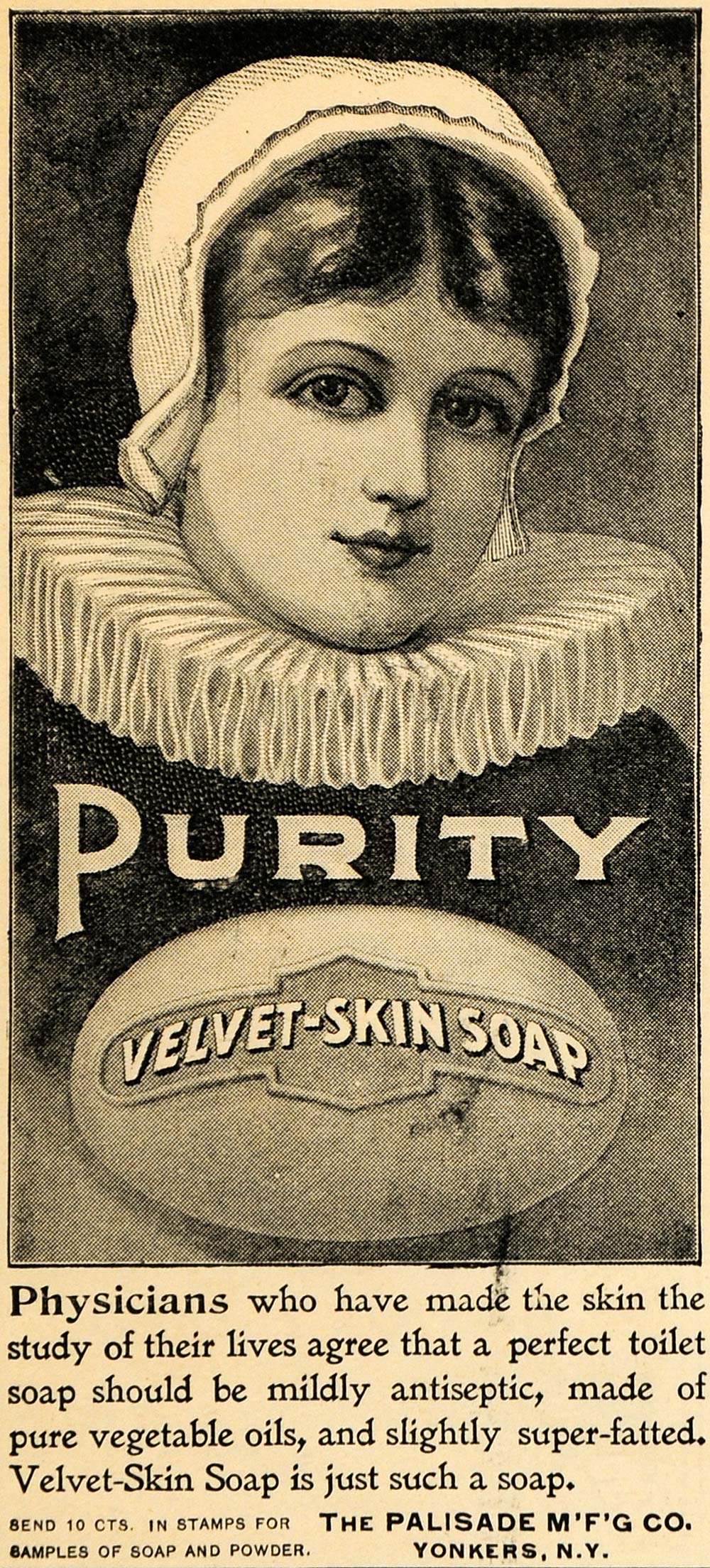This vertical black and white vintage advertisement, likely from the early 20th century, features a detailed illustration of a woman wearing a white bonnet and a highly ruffled, pleated Victorian-style collar. Her expression is a mildly content, neutral look. Beneath her image, the word "Purity" is prominently displayed in an antique-style font. Just below lies a logo revealing a bar of soap labeled "Velvet Skin Soap." The text further promotes the soap's quality, stating: "Physicians who have made the skin the study of their lives agree that perfect toilet soap should be mildly antiseptic, made of pure vegetable oils, and slightly super-fatted. Velvet Skin Soap is just such a soap." At the bottom, the advertisement instructs readers to "Send 10 cents in stamps for samples of soap and powder," and credits the product to the Palisade Manufacturing Company, Yonkers, New York. The overall layout and detailed description hint at its period authenticity, reflecting its likely origin from a magazine or newspaper.